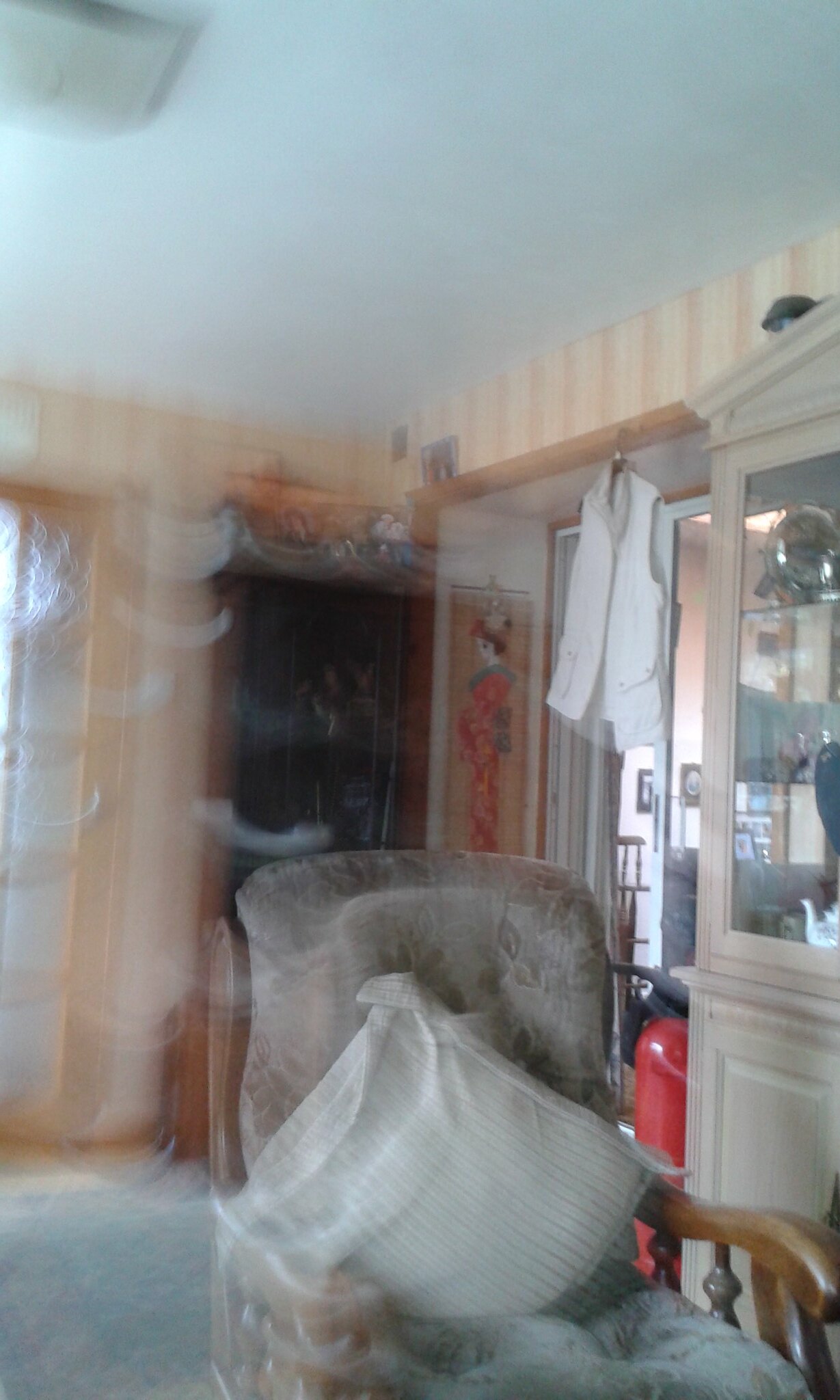The photograph captures a cozy living room with intricate details. Central to the image is an upholstered chair featuring a brown wooden frame and curved arms, adorned with a floral cream cushion and a large white pinstripe pillow. The backdrop showcases striped walls in cream and pale orange hues, adding warmth to the space. On the right side, a light blonde wood china cabinet stands elegantly, displaying various items on its glass shelves, including a notable gold clock on the top shelf. The white ceiling provides a clean contrast to the room’s decor. The back wall features an Asian Japanese art piece, contributing a cultural touch. Above an archway that leads to another room, a white vest is casually hung, adding a personal and lived-in feel to the scene.